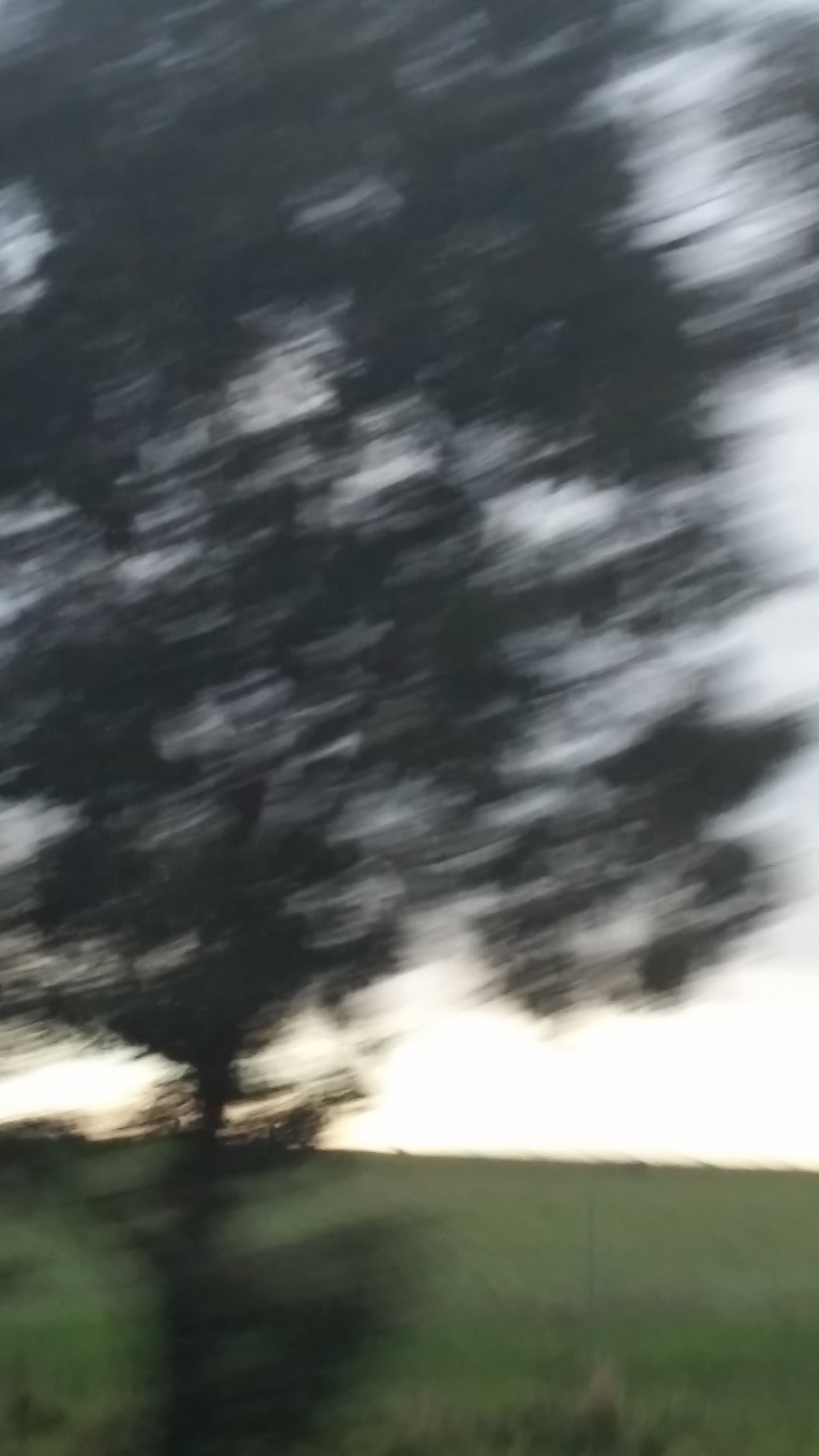Captured from a moving vehicle, this image reveals a blur of motion, featuring a prominent dark green tree occupying the lower right-hand side of the frame. The tree's foliage extends upwards, taking up approximately two-thirds of the picture, while the remaining portion is a mix of green grassland and a white, overcast sky, hinting at a sunny yet overcast day. The lush green grass suggests a gentle hill, and there appears to be a faint outline of a fence, though it's difficult to discern due to the blurriness. The sense of motion is palpable, enhancing the transitory nature of this countryside scene.